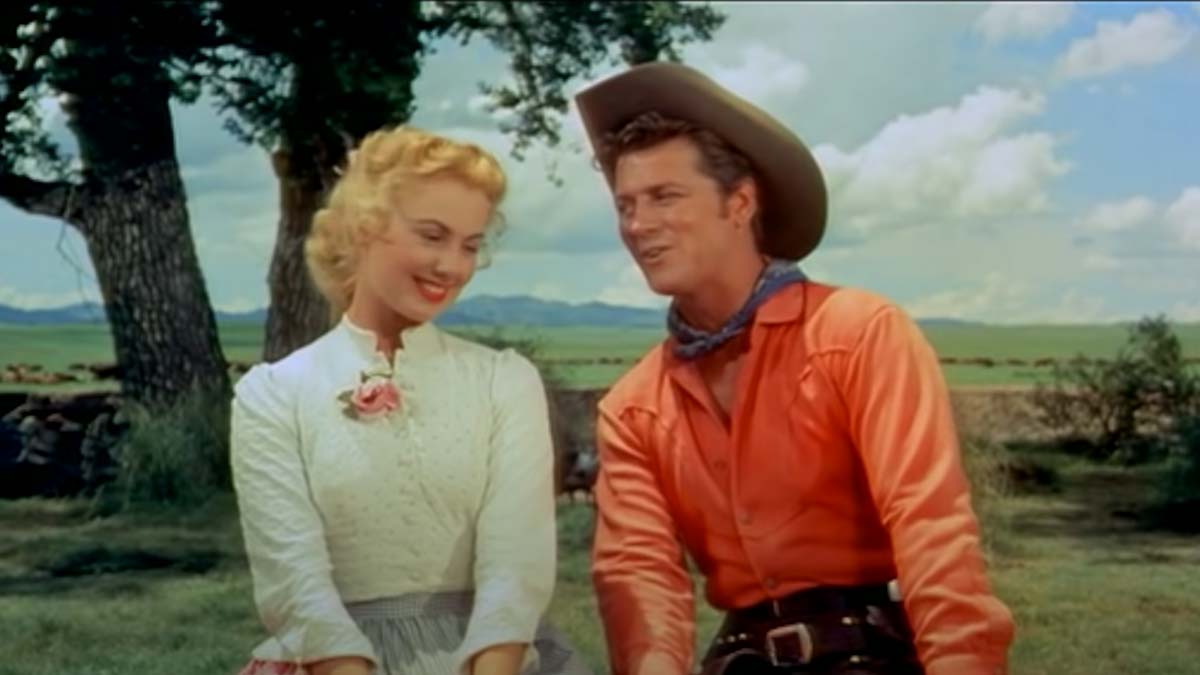In this vivid scene from the country movie "Oklahoma," Ado Annie, a woman in her late 20s with short, curly blonde hair tied in an updo, sits smiling with her head turned slightly to the right. She is dressed in a white ruffled button-up shirt adorned with a pink flower or rose brooch and a blue skirt. Beside her, leaning in closer as if in conversation, is Will Parker. Will is depicted wearing a reddish-orange long-sleeve button-up shirt, black pants, and a blue bandana tied around his neck. He completes his cowboy look with a brown hat and a pair of guns at his hips. The background showcases a serene landscape featuring green grass, two distinct trees, distant mountains, and a sky filled with white clouds. Both characters are seated attentively, capturing a moment of charming interaction, set against a picturesque pastoral backdrop.